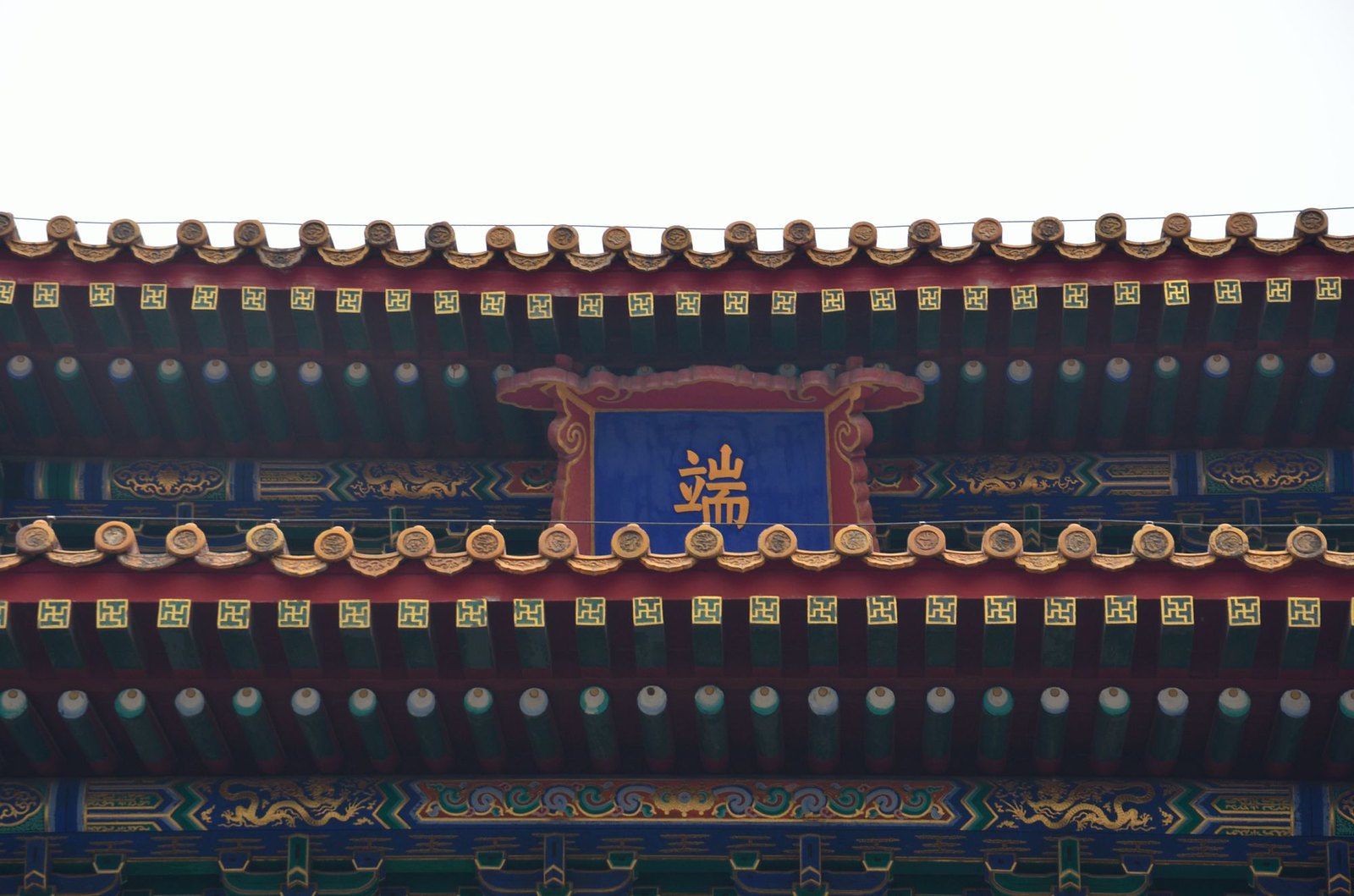The image showcases an ornate, recently renovated rooftop of a traditional Chinese structure. The intricate wooden architecture features support solely from its elaborately carved wood without any visible metal elements. The primary color palette consists of yellow, red, and blue, accentuated by detailed depictions of dragons and mythological beasts that adorn the rooftop. The design is heavily patterned with repeating shapes including circular motifs, square bars, and meticulously placed rods, creating a sophisticated and busy appearance. Central to the composition is a wooden plaque with a blue background, prominently displaying a golden Chinese character. This plaque is bordered by an exquisitely detailed frame, contributing to the overall vibrant and colorful aesthetic, with touches of gold, green, and hints of other vibrant colors interspersed throughout the structure.